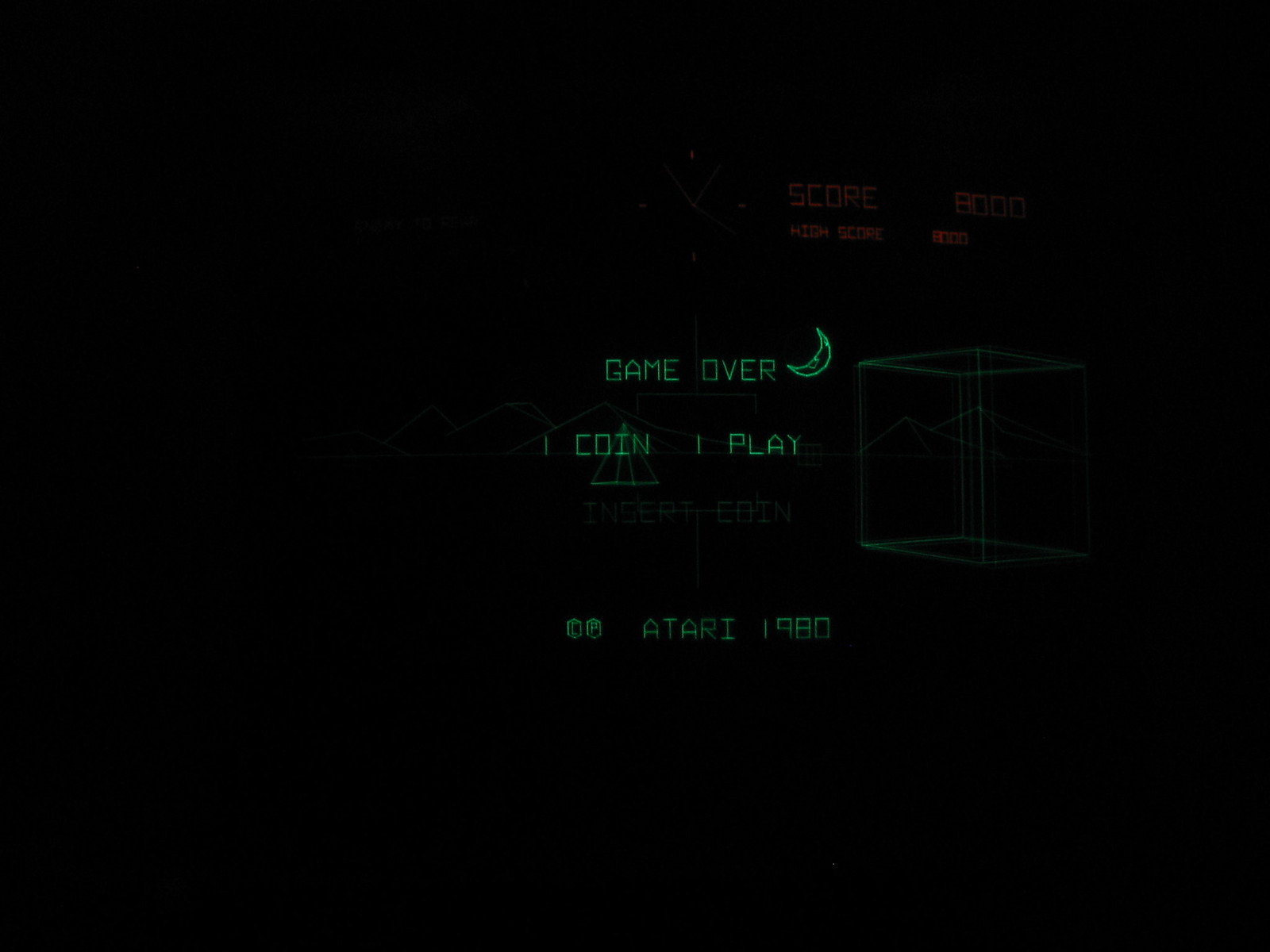A dimly lit screen capture reminiscent of classic Atari video games. The screen primarily consists of a black background, punctuated by simple, green graphics characteristic of early 1980s game design. At the center, the phrase "Game Over" appears in thin green print, accompanied by a crescent moon symbol. Below the main text, a smaller message reads "One coin one play," inviting players for another round. In the lower middle section, "© Atari 1980" indicates the game's vintage origins. Scattered across the display are faint horizontal lines, adding to the nostalgic, retro atmosphere of the image.